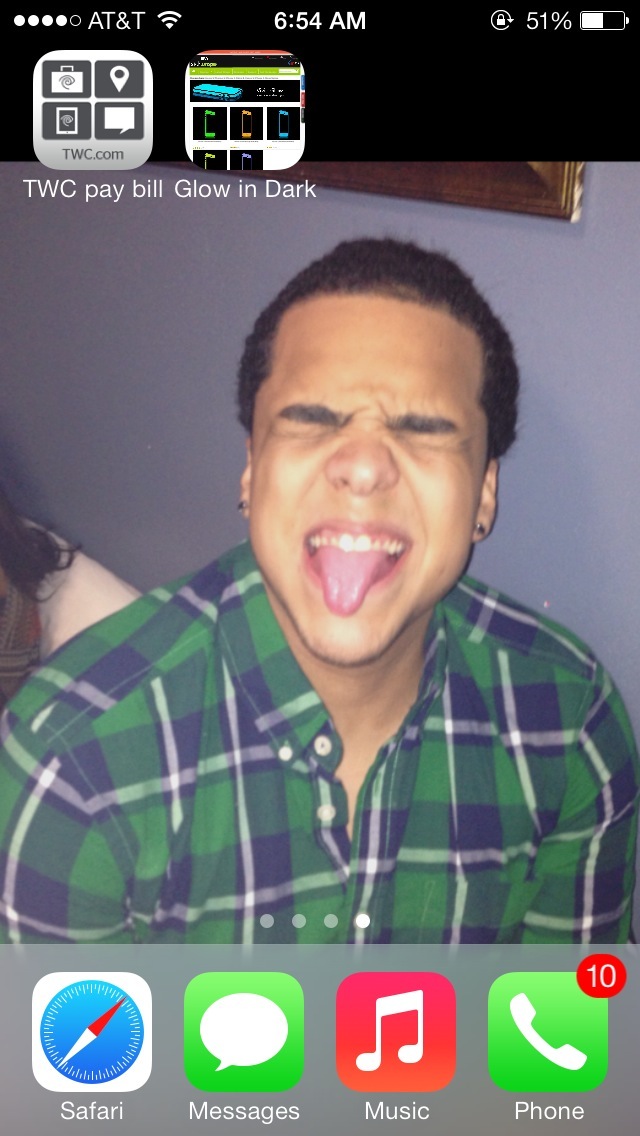The image is a screenshot of an iPhone home screen featuring a young man with slightly curly hair wearing a blue, green, and white plaid shirt. His eyes are clenched shut, and he is sticking out his tongue. The man, who also wears earrings, is sitting in front of a purplish wall. The iPhone indicates it's 6:54 a.m., connected to AT&T with a Wi-Fi signal, and has 51% battery remaining. Several details in the status bar include the time, the battery icon, and phone signal bars. Beneath the wallpaper, the home screen displays icons for Safari, Messages (with 10 missed notifications), Apple Music, and the Phone app, all in different colors. Text icons at the top of the screen show "TWC.com," "TWC pay bill," and "glow in the dark."